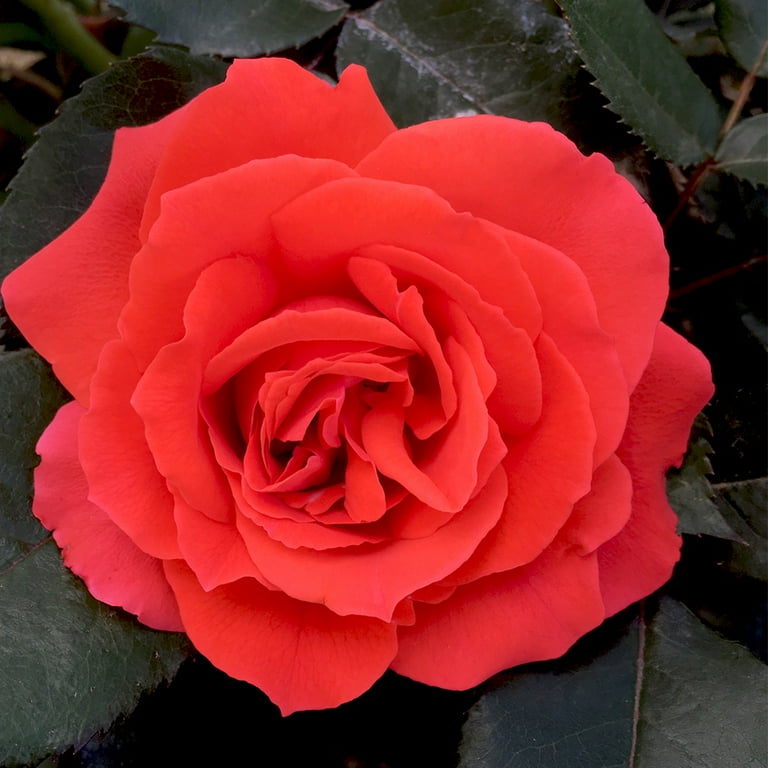This close-up photograph features a captivating, large rose in full bloom, dominating the square frame with its vibrant, deep red petals. The intricate folds and layers of the petals are meticulously detailed, creating an engaging sense of depth and movement. The rose, unusual in its intensely dark yet bright color, suggests the image may have been taken in shaded lighting or enhanced with a filter. Surrounding the rose are thick, substantial dark green leaves characteristic of a rose bush, adding to the dramatic contrast and making the vivid flower the focal point of the image. The captivating beauty of the perfectly bloomed rose against the lush, dark green foliage creates a visually striking and immersive scene.